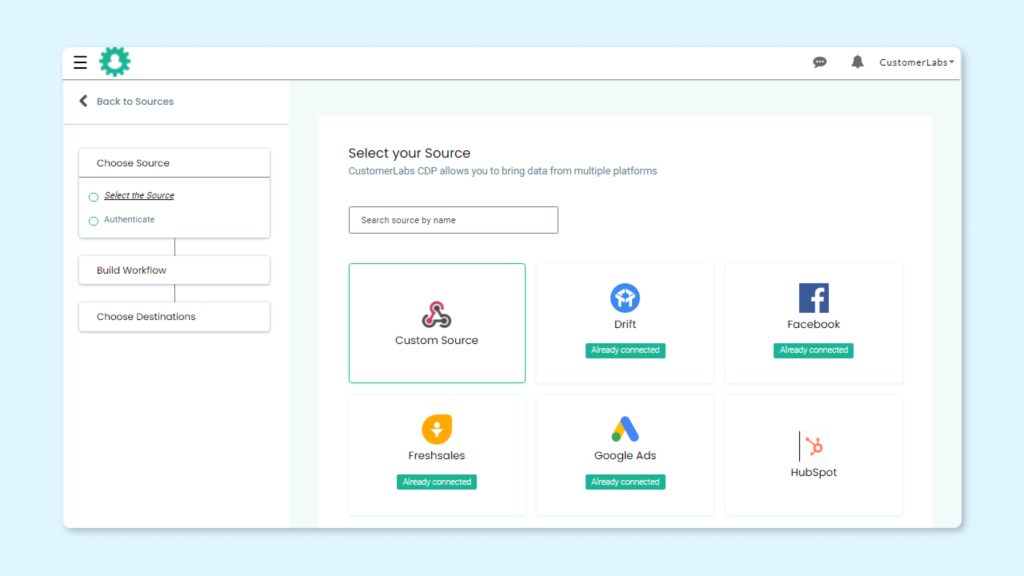This image, captured from a device screen, features a web page with a predominantly light blue background that transitions to white in the central area. The central section, slightly tinged with greenish-gray in one area, displays the heading "Select Your Source." Beneath this heading, the text "Customer Labs CDP allows you to bring data from multiple platforms." is prominent. Below this statement is a rectangular search bar labeled "Search source by name."

Underneath the search bar are six clickable rectangles arranged in two rows. The first rectangle, labeled "Custom Source," is followed by "Drift," which has a green box underneath indicating "Already Connected." Next, "Facebook," featuring the iconic "F" logo and similarly marked by a green "Already Connected" box.

In the second row, "Freshsales" and "Google Ads" both display green "Already Connected" tags. The last rectangle is labeled "HubSpot," which does not have a connection status displayed.